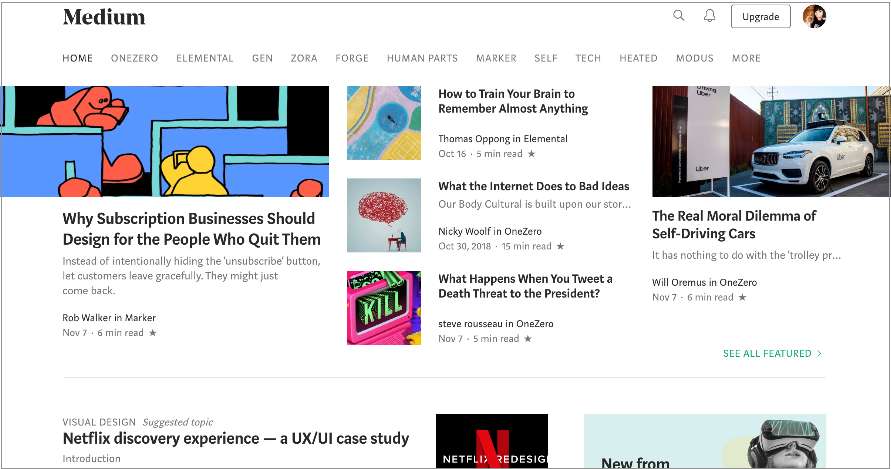This is a screenshot taken from a computer screen displaying the Medium website. At the top, the Medium logo is prominently displayed with a capital "M". Directly below the logo, there is a navigation bar with clickable sections. The sections listed in order are: "Home," followed by "1-0" (one-zero), "Elemental," "Gen," "Zora," "Forge," "Human Parts," "Marker," "Self," "Tech," "Heated," "Modus," and "More." Above the "More" section, there are icons for a magnifying glass (search function), a bell (notifications), an "Upgrade" button, and a circular profile picture.

As you look further down the page, on the left side, there is an image featuring shades of blue, teal, orange, and yellow. The image appears to depict people working in cubicles. Below the image, there is a headline that reads: "Why subscription businesses should design for the people who quit them."